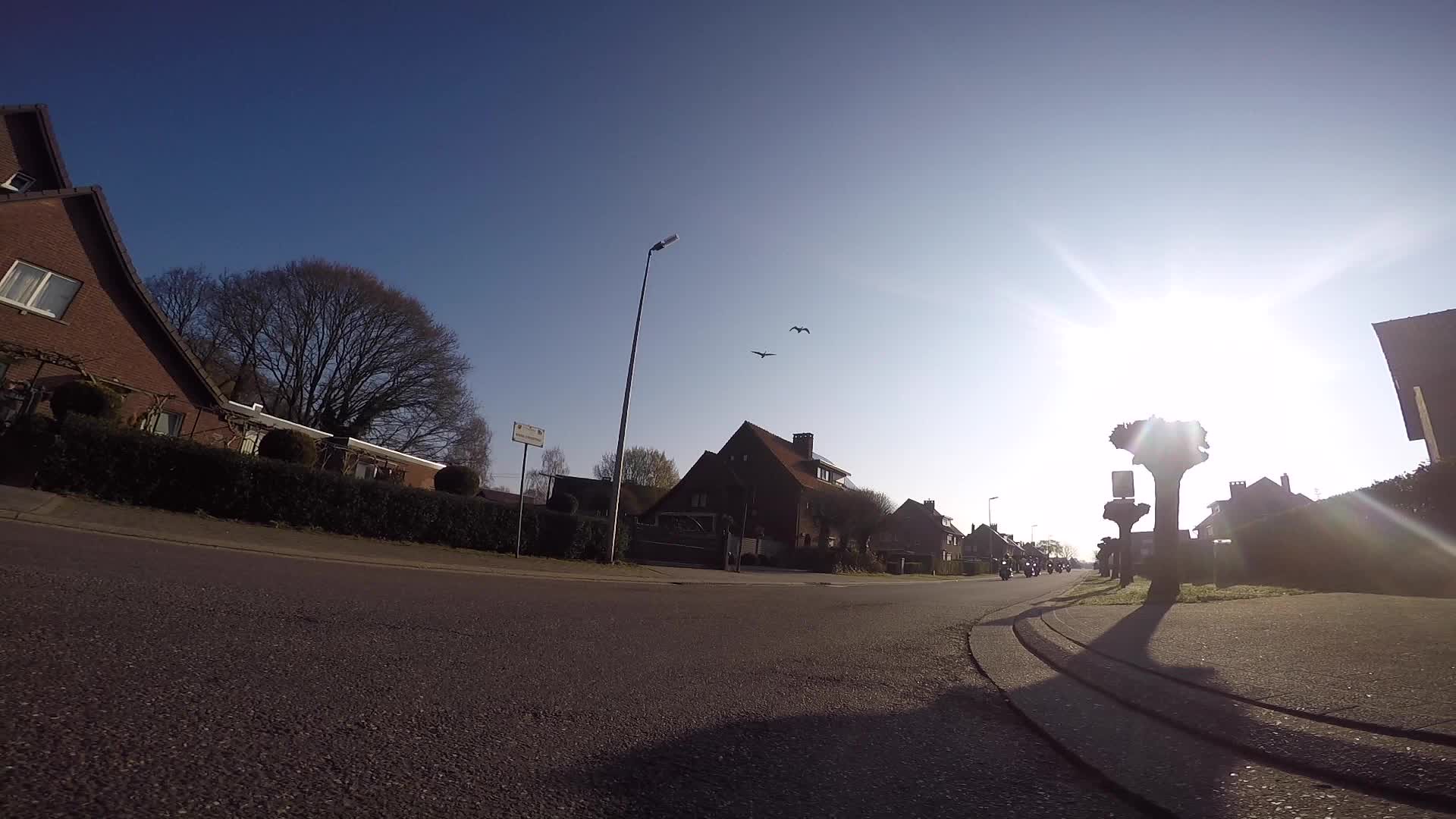This photograph captures a serene residential neighborhood, taken from a low angle as if the camera was placed directly on the road surface. The perspective allows a slightly upward view, showcasing the street and the spacious homes that line it. These houses, all uniformly dark brown with brownish-red roofs, add a cohesive and warm aesthetic to the scene. On the right side of the image, a prominent, round sunburst effect suggests the presence of the sun, creating a dramatic illumination that enhances the atmosphere, although it doesn't distinctly indicate sunrise or sunset.

The sky above is a striking bright blue, adorned with a pair of birds in flight, adding a touch of liveliness to the tranquil setting. Additionally, the street is accented with street lights and various street signs, which contribute to the urban landscape. In the foreground, a line of motorcycles is seen rounding the corner, infusing a sense of motion and subtle dynamic energy into the otherwise still and peaceful environment.